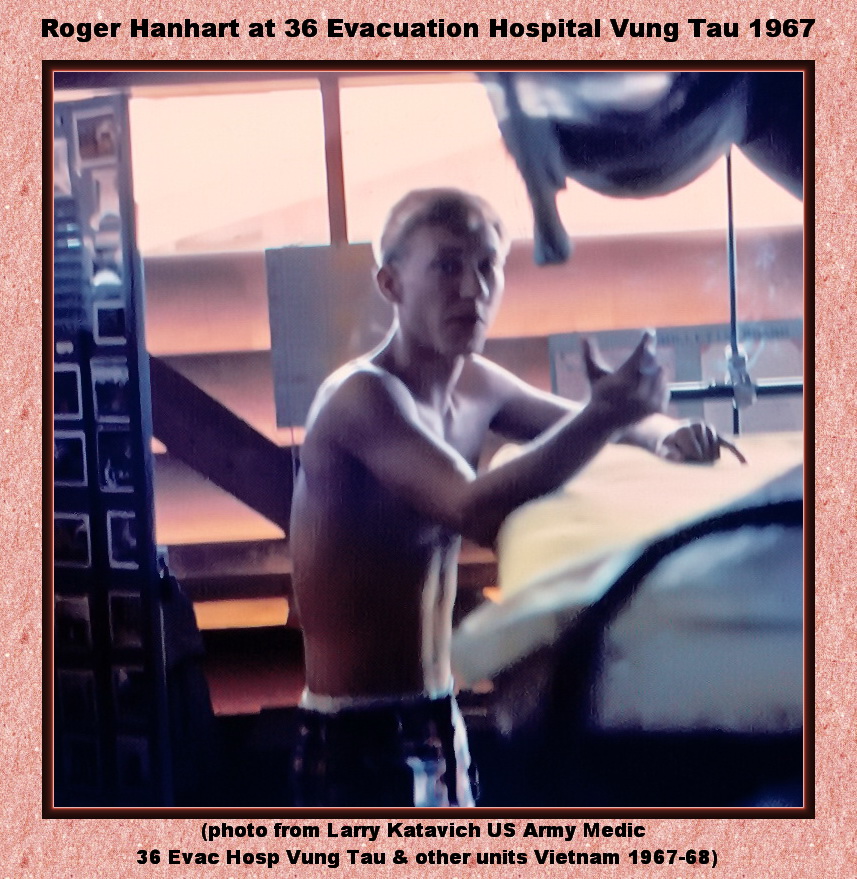This vintage photograph from 1967 depicts a shirtless young man, likely in his early twenties, with blonde hair, standing amidst an indoor setting that seems to resemble either a barracks or a hospital room, possibly within the 36th Evacuation Hospital in Vung Tau, as indicated by the captions. The man is looking directly at the camera and making a gesture with his hands. He is wearing military-style pants that are slightly sagging, revealing his white underwear. The background is somewhat ambiguous, featuring elements such as a glass window, a white sheet, and what appears to be metal objects or bunk beds. There is a smokey or hazy quality to the image, giving it a reddish tint, which adds to its vintage feel. The photograph is square-shaped with a dark brown border, surrounded by a wider pink border with inscriptions. The top of the frame reads, "Roger Hanhart at 36th Evacuation Hospital, Vung Tau, 1967," and the bottom states, "Photo from Larry Katowicz, U.S. Army medic, 36th Evac Hospital, Vung Tau, and other units, Vietnam, 1967-68." Despite some blurriness and difficulty in identifying all elements in the room, the photo effectively captures a moment in time for Roger Hanhart at the evacuation hospital.